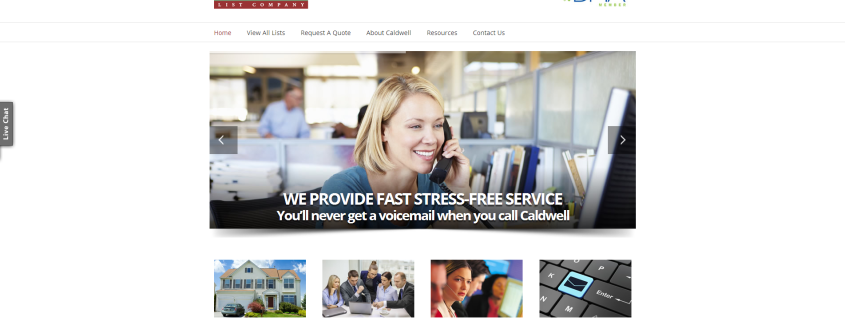Image Description: 

The image prominently features a woman in an office setting, holding a phone and looking at a computer screen. Behind her, a man is also present, engaged in a background activity. At the very top of the image, there is a small, reversed print text "Liz Comedy" in white against a red box. 

The primary focus of the computer screen appears to be a website displaying a variety of real estate or service options. The header on the screen contains several navigation links: "Home," "View All," "Request a Quote," "About Caldwell," "Resources," and "Contact Us," all set against a predominantly white background with a specific home page in red.

To the left of the woman, there is a live chat option described as "You Talk, We Listen" inscribed vertically in grey. Surrounding this woman are various navigable images indicated by arrows positioned to her left and right, allowing users to cycle through them.

Beneath this main section are four thumbnail images, each depicting different scenarios: 
1. A massive beige two-story home with numerous windows and a parked car, surrounded by shrubs.
2. A group of people in an office setting intently looking at a computer screen and pointing.
3. A woman with a headset on, appearing to be concentrating on something, with other colleagues nearby.
4. A close-up shot of a keyboard with a glowing blue icon resembling a male figure, possibly symbolizing an email or messaging service.

The overall theme suggests providing fast, stress-free services, emphasizing that customers will never receive a voice call, specifically when interacting with Caldwell's services. The clean and functional layout, paired with the diverse imagery, underscores a professional and efficient service experience.